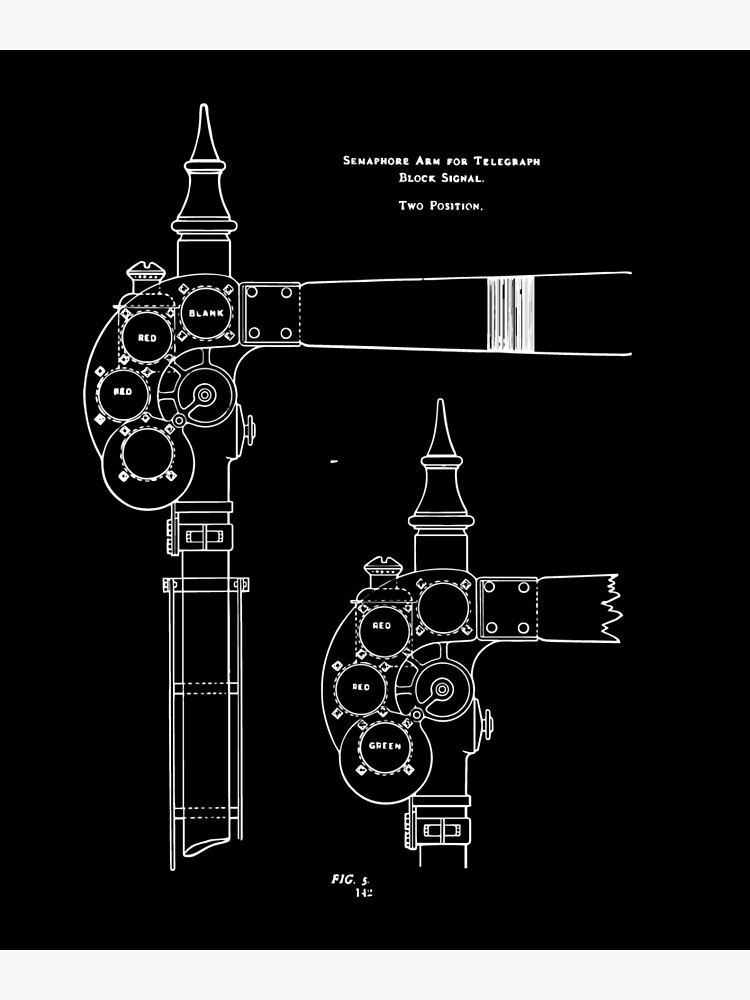This image is an intricate technical illustration set against a black background with white text and lines. It prominently features the label "semaphore arm for telegraph, block signal to position" at the top. The illustration consists of two detailed diagrams of a semaphore arm. 

The primary diagram on the left depicts a complete semaphore arm with a decorative finial at the top of a vertical post. Attached to this finial is a curved mechanism displaying various labeled dials or buttons. The upper part includes labels for "blank," "red," and "red." Below this, a detailed cutaway of the same mechanism shows additional labels for "red," "red," and "green," with rounded surfaces and rectangular extensions highlighted.

The smaller inset diagram beneath the main one provides further detail, focusing on the upper left section of the semaphore arm, showing a similar arrangement of dials. This inset illustration appears to be a close-up, revealing intricate elements not fully expanded in the main drawing. At the very bottom of the illustration, the text "figure 5, article 112" and "figure 5142" are noted, indicating its reference within a larger document.

Overall, the image emphasizes the functional and structural components of the semaphore arm, with clear demarcation of its signal positioning system.